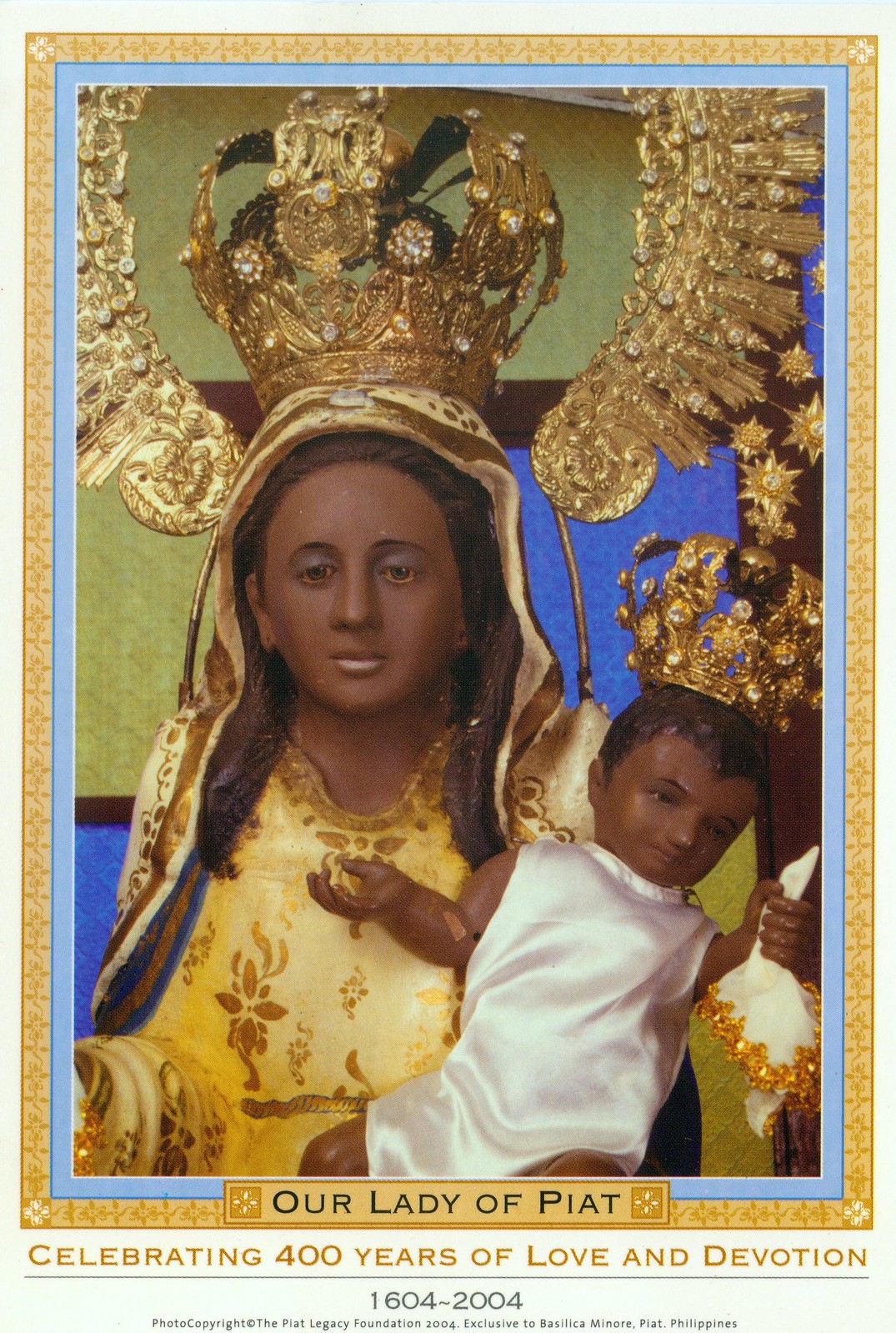This is an elaborate, colorful drawing of Our Lady of Piat, titled "Our Lady of Piat" at the bottom, with the inscription "Celebrating 400 Years of Love and Devotion 1604 to 2004." The image depicts a dark-skinned woman with long brown hair and halfway-closed eyes, donning a gold dress, robe, and an ornate golden crown adorned with almost feather-like gold decorations. She wears a gold veil on her head and a touch of light blue eyeshadow. The woman cradles a similarly brown-skinned baby in her left arm, who is dressed in a luxurious white satin gown and holds a white handkerchief with golden edges. The baby, possibly a boy, also wears a large crown, suggesting royal status. Golden stars accentuate the image, adding to its sacred and celestial feel. The woman's facial expression conveys rigidity, and she appears almost statue-like within a gold-bordered frame, characteristic of Catholic holy cards venerating saints.